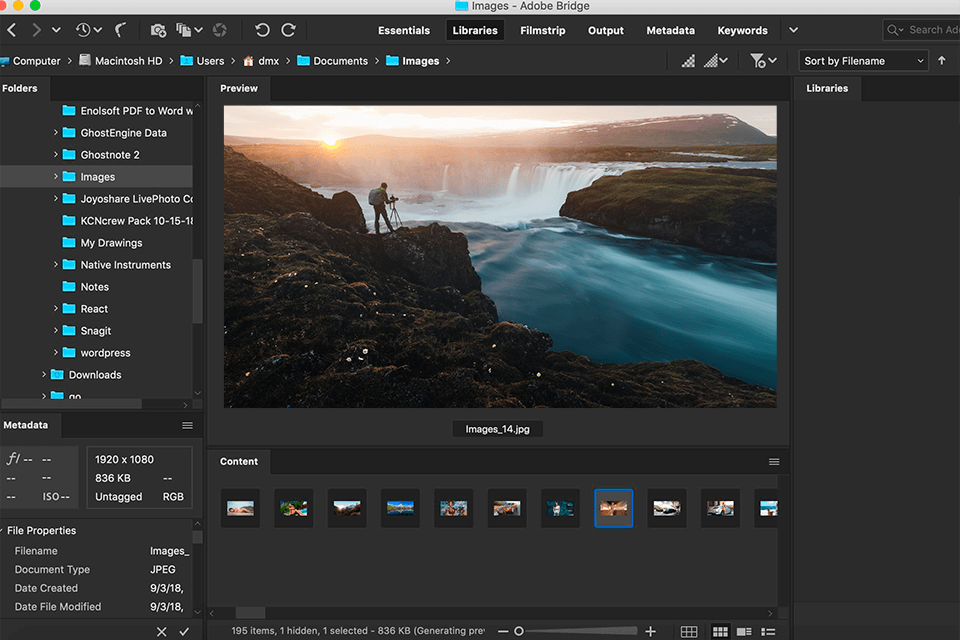Here’s a cleaned-up and detailed caption:

"A straight-on view of a computer screen displaying Adobe Bridge's 'Images' section. The user is viewing a stunning landscape photograph, which takes center stage on the screen. The image depicts a person standing amidst a vast, hilly, and mountainous terrain, surrounded by cascading waterfalls and a crystal blue body of water flowing through the scene. The sun can be seen reflecting off the water in the picture, adding a luminous glow from the horizon. The interface shows that the user has navigated to the 'Images' section on the left sidebar, bringing this picturesque photo into focus on the main display."